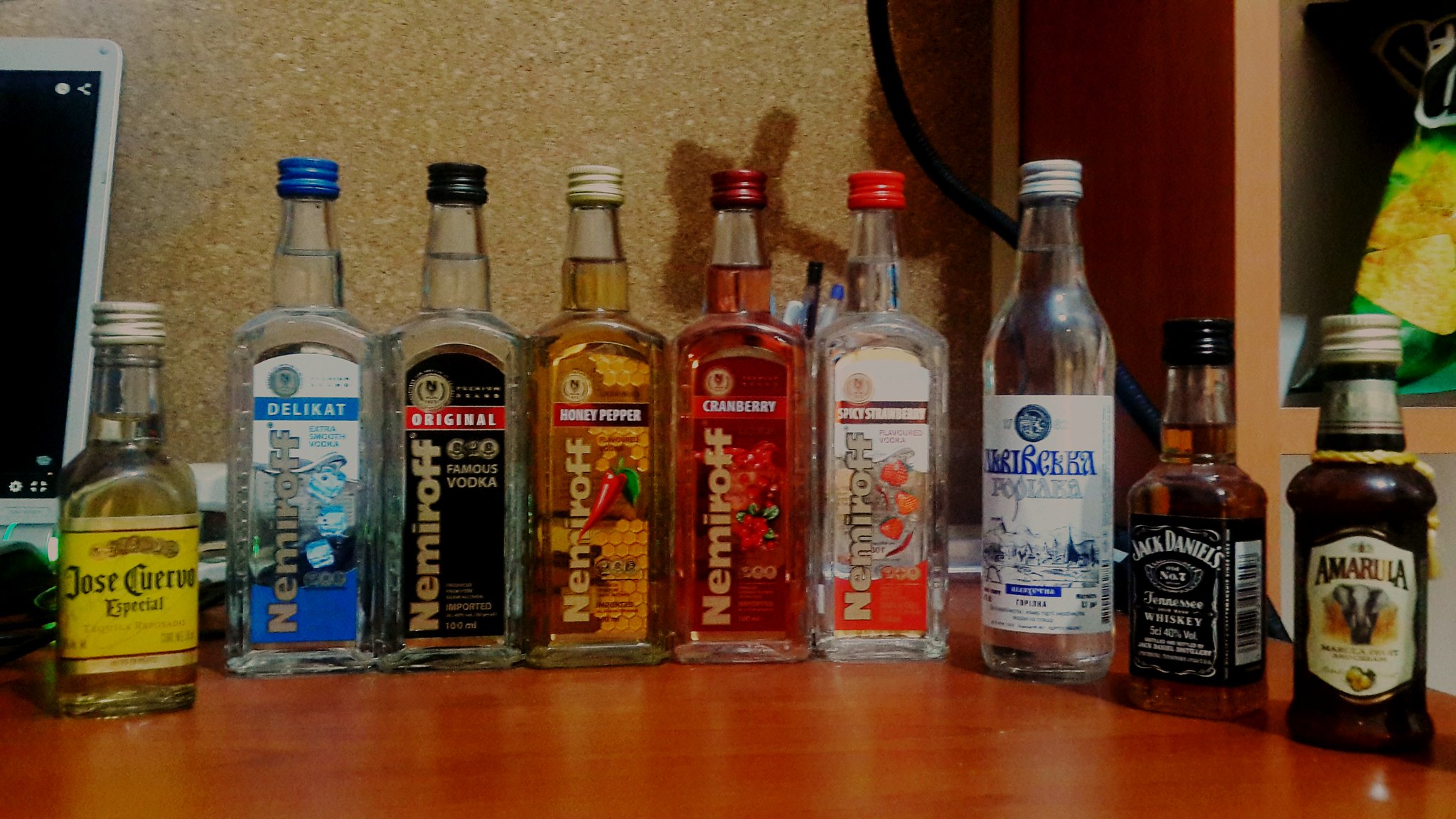This image displays a cherry wood desk lined with an array of alcoholic beverages. The lineup forms a slight curve, showcasing a diverse collection with notable emphasis on Nemerov vodka, which appears in multiple flavors. The first bottle on the right is a full bottle of Jose Cuervo Especial, distinguished by its yellow label and silver top. Next is a bottle of Nemerov Delicate Citrus Smooth vodka, featuring a blue label with silver writing and an image of blue ice cubes.

Following that is a bottle of Nemerov Original vodka, which has a striking black label with a red top banner that reads "Original" and vertical gold writing. Adjacent is Nemerov Honey Pepper vodka, marked with a honeycomb design and a pepper graphic intersecting the label. The line continues with Nemerov Cranberry vodka, evident from the cranberries depicted on the left side of the bottle and a white "Cranberry" banner.

Further down is Nemerov Spicy Strawberry vodka, characterized by a shiny red banner and strawberry imagery. Another bottle with an unclear name but a white label and blue writing, possibly another vodka, follows this. Then, a smaller bottle of Jack Daniel's Tennessee Whiskey adds to the assortment with its familiar black label and white writing.

The last bottle is Amarula, easily recognized by its dark appearance, silver top, and a hanging tag. The scene suggests preparations for a social event, with the edge of an open laptop visible on the left and a faint glimpse of a computer monitor on the right, adding to the context of a modern, casual gathering space.